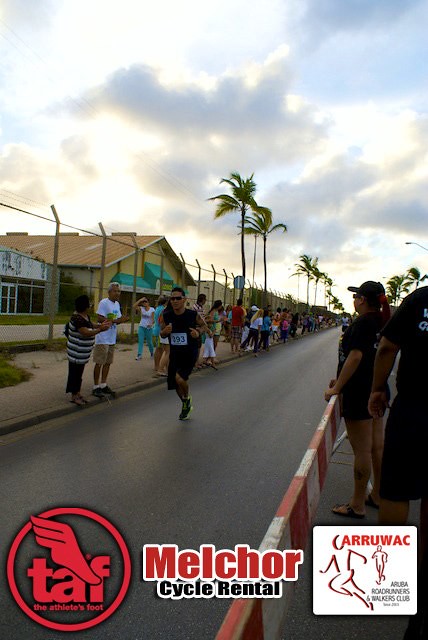The image appears to be an advertisement or promotional flyer featuring a road running event sponsored by Melchor Cycle Rental, The Athlete's Foot, and the Carawack Aruba Roadrunners and Walkers Club. The main scene captures a single runner, prominently numbered 393, clad in a black t-shirt and shorts with bright green-soled training shoes, making his way down a sunlit road. He is flanked on one side by a tall chain-link fence topped with barbed wire and spectators standing on a sidewalk behind it. Additional people can be seen behind temporary red and white barriers lining the road, cheering on the participants. In the backdrop, there are palm trees, various properties, and buildings. The vibrant setting suggests it's later in the afternoon with the sun lowering behind light, scattered clouds. Logos for the sponsoring organizations are visible in the corners of the image, including a red winged foot symbol and the letters "TAF" for The Athlete's Foot, alongside inscriptions for Melchor Cycle Rental and the Carawack Aruba Roadrunners and Walkers Club.